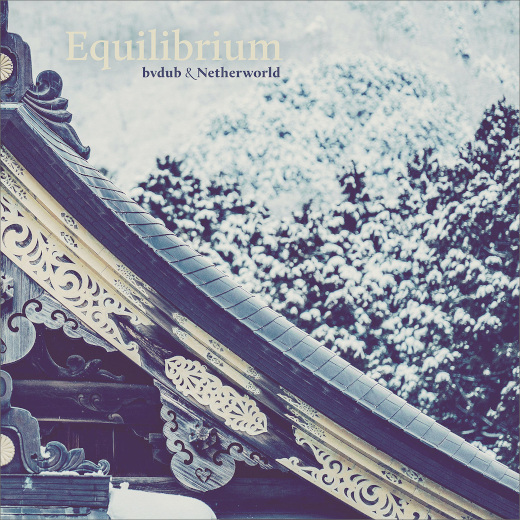The square-shaped image appears to be an artfully designed background reminiscent of a CD cover or textbook. It prominently features the word "equilibrium" in a cream color at the top left, with "BV Dub and Netherworld" in a smaller, grayish-blue font underneath. The image itself has a predominantly light cream to grayish-blue color scheme with some darker elements and a washed-out aesthetic. The top half of the picture is split diagonally from left to right, revealing an abstract sky and tree foliage on the right side. The bottom half displays an intricate, ornate design of a building’s awning, roof, or archway, with lighter curlicue patterns against a darker background. The image is marked by a detailed, cream-colored border design on the inside, creating a sense of depth and complexity. The middle trimming of the roof features a darker section that may be painted arrows, further adding to the overall artistic feel of the image.